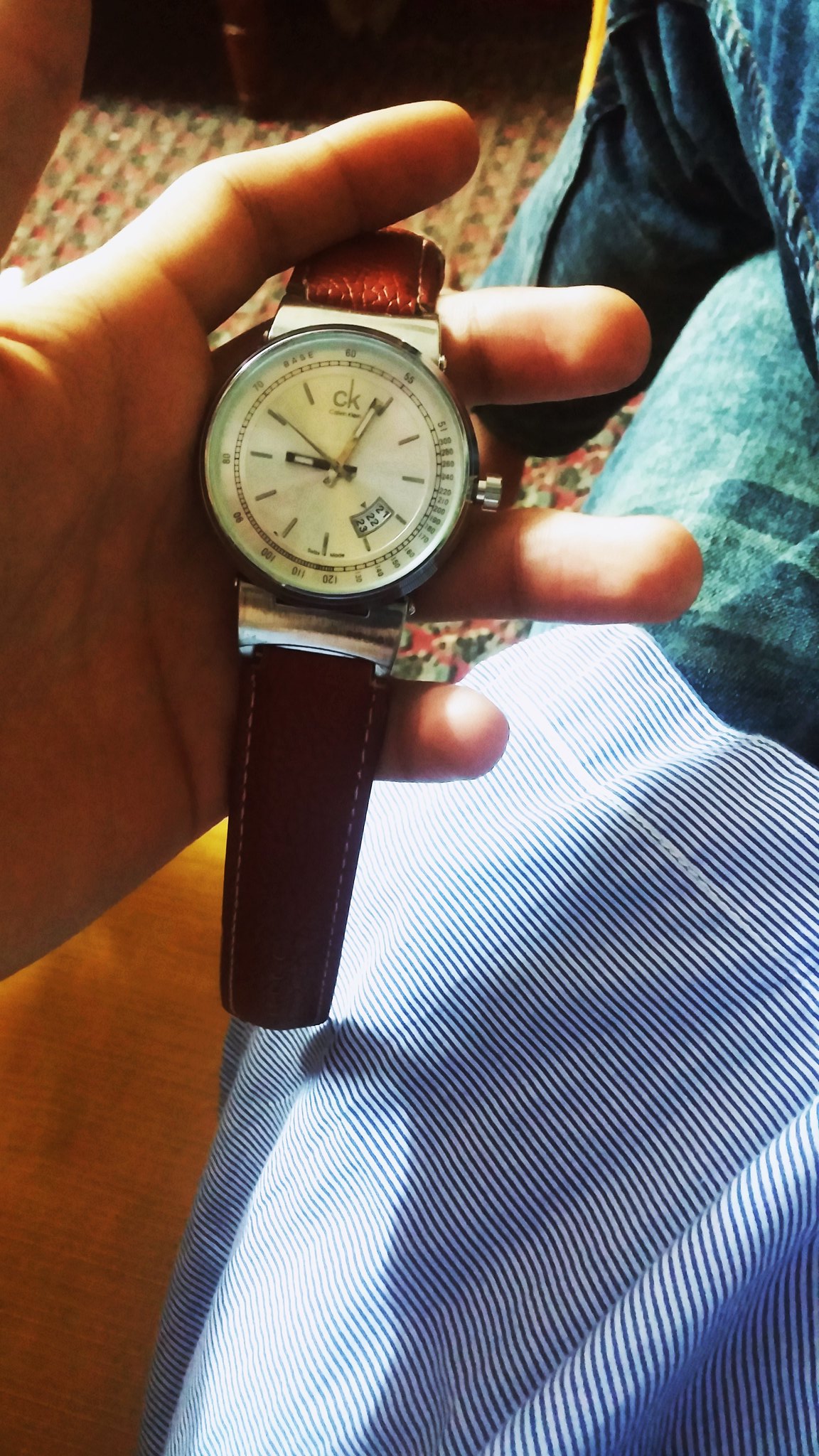A point-of-view photograph captures a person wearing blue denim jeans and a blue and white striped shirt, holding a wristwatch in their outstretched left hand. The watch features a brown leather band with silver clips and a white face. The face displays gold hands and lines representing each number, along with a CK logo at the 12 o'clock position. A wooden floor is visible on the left side and in the background, there's a textured brown and beige rug. The watch also includes a silver circular border around its face and possibly a small window for additional details. The photo appears to have been taken using a cell phone in portrait mode.